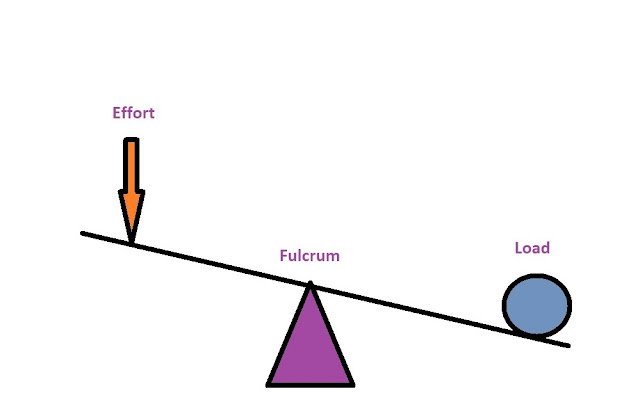The image is a simple scientific diagram set against a white background. At the center, there is a purple triangle outlined in black, labeled "fulcrum" in purple font at its apex. Resting on the triangle is a black line, resembling a teeter-totter, inclined downwards to the right. An orange arrow, labeled "effort" in purple font, touches the line on the elevated left side, while a bright blue circle, labeled "load," sits on the lower right side. The diagram clearly illustrates a basic physics principle despite the lack of additional explanatory text.